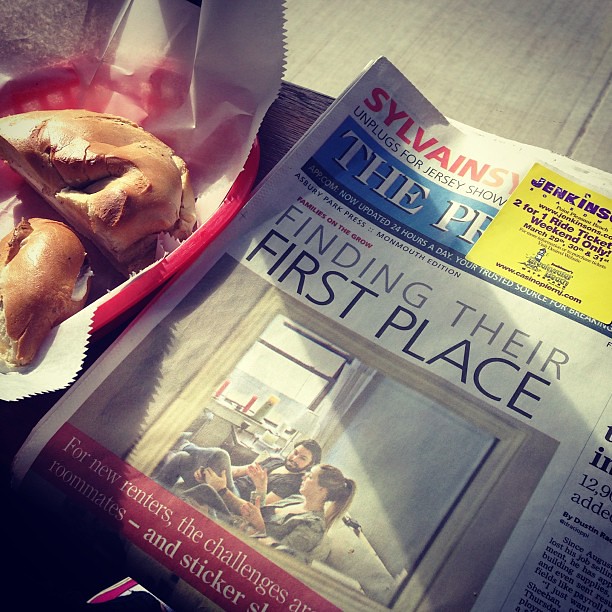The image portrays a detailed scene featuring a newspaper and a sandwich. In the upper left corner, there is a brown bagel sandwich cut in half, placed within a red basket lined with white paper. The foreground is dominated by the front page of a newspaper, slanted and laying against a table with the bottom right corner visibly distinguishable. The headline of the newspaper reads "Finding Their First Place," and it includes an image of a girl and a man sitting on a white sofa, with a cityscape through a window behind them. The overall color palette includes shades of gray, white, red, light brown, maroon, pink, blue, yellow, and purple. Additional articles and banners on the newspaper include "Sylvain," “Lynn Plugs for Jersey Show”, "The PR," and a yellow sticker mentioning “Jenkins’ Two-for-One Ride Today, Weekend Only.” Judging by the ambient lighting, the setting could be outdoors in the middle of the day, possibly in a restaurant or someone's kitchen.